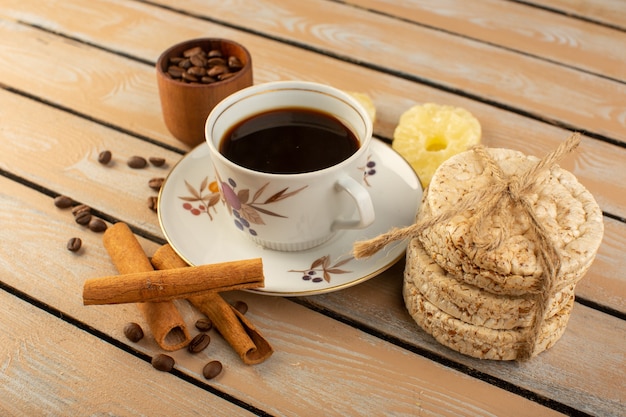The image showcases a serene, rustic coffee setting on an outdoor, diagonally-aligned, wooden table. At the center of the table is a white coffee cup with a matching saucer, both adorned with a floral pattern featuring hues of brown, red, yellow, taupe, and blue. The cup, filled with dark black coffee, has a gold rim around its inner lip and a handle facing slightly forward and to the right. The saucer also features a similar floral pattern with additional, delicate details suggesting brown wheat husks and berries. The coffee setup is accompanied by various elements: to the left of the cup, there's a cluster of coffee beans and three cinnamon sticks arranged in a slight diagonal pattern. Behind the cup, a small brown container filled with coffee beans adds texture and depth to the composition. To the right, a stack of three rice crackers snugly tied with a tan twine bow provides an element of rustic charm. Additionally, behind the saucer, two stacks of dried pineapple rings lend an extra touch of visual and textural interest. The table itself, with its white and peach-stained wooden boards showcasing visible wood grain, further enhances the cozy, country-style ambiance of the scene.